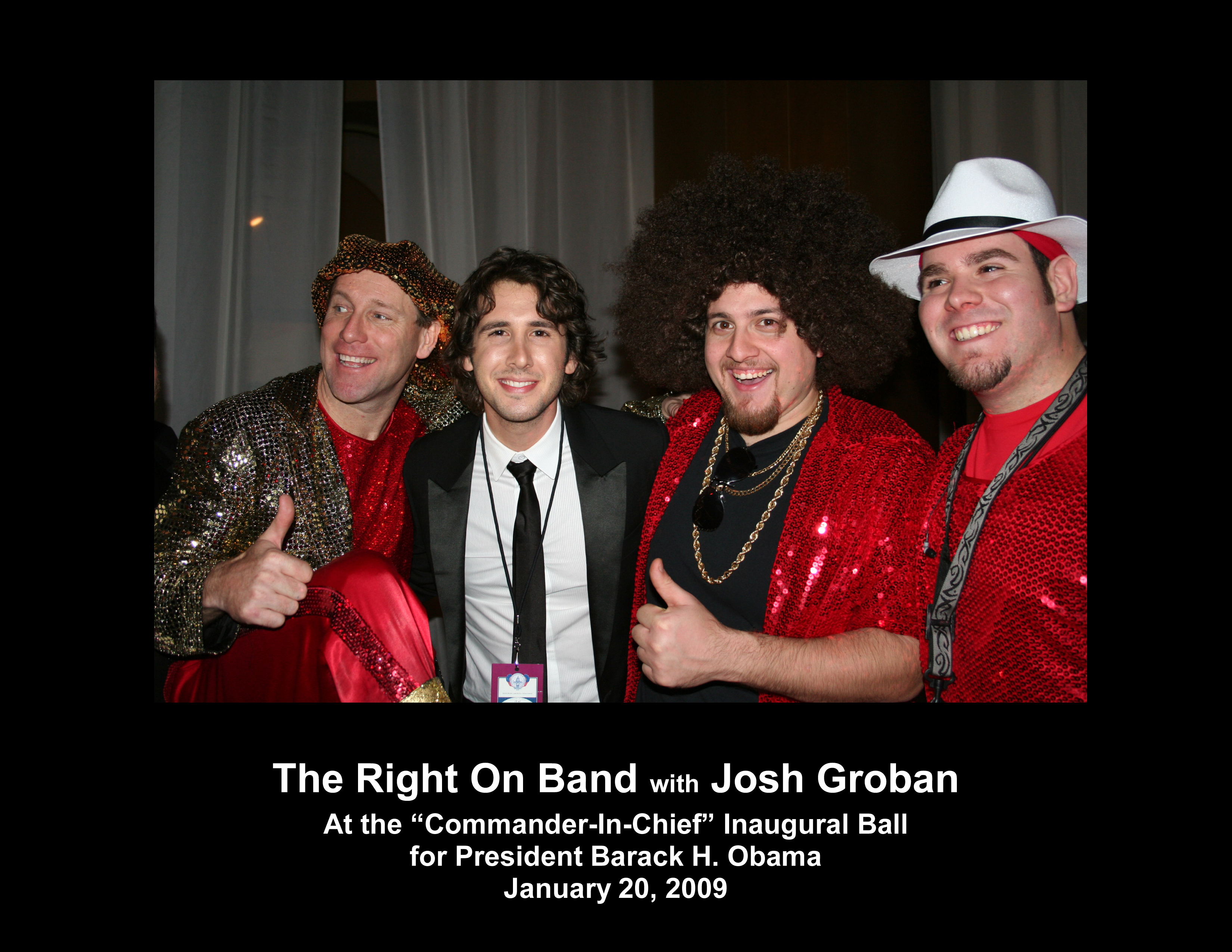In this vibrant color photograph, four men, including singer Josh Groban, pose together against a backdrop of white curtains. The man on the far left is a white male adorned in a striking brownish-gold sequined hat, a shimmering black sequined jacket, and a red sequined shirt. He exudes flair with satin red pants edged with sequins, gold sequined boots, and a thumbs-up gesture from his right hand while lifting his right leg.

Next to him stands Josh Groban, a white male with dark hair, donning a polished look with a white button-down shirt, black tie, and a tuxedo jacket featuring large lapels. He wears a name tag necklace with a purple, blue, and white badge on a black rope and smiles warmly at the camera.

Beside Josh is another white male, characterized by his thick dark curly hair and robust beard. He sports a black t-shirt accentuated with gold chains, black sunglasses dangling from the shirt, and a red sequined short-sleeved shirt. His left hand mirrors a thumbs-up gesture.

On the far right, another white male completes the group, distinguishable by his white hat with a black band. He is clad in a red sequined shirt and a black and silver band necklace, complemented by a goatee.

The radiant outfits and cheerful expressions of the men, coupled with the elegant white curtains in the background, capture the celebratory ambiance of this moment. At the bottom of the image, white text reads: "The Right On Band with Josh Groban at the Commander-in-Chief Inaugural Ball for President Barack H. Obama, January 20, 2009."